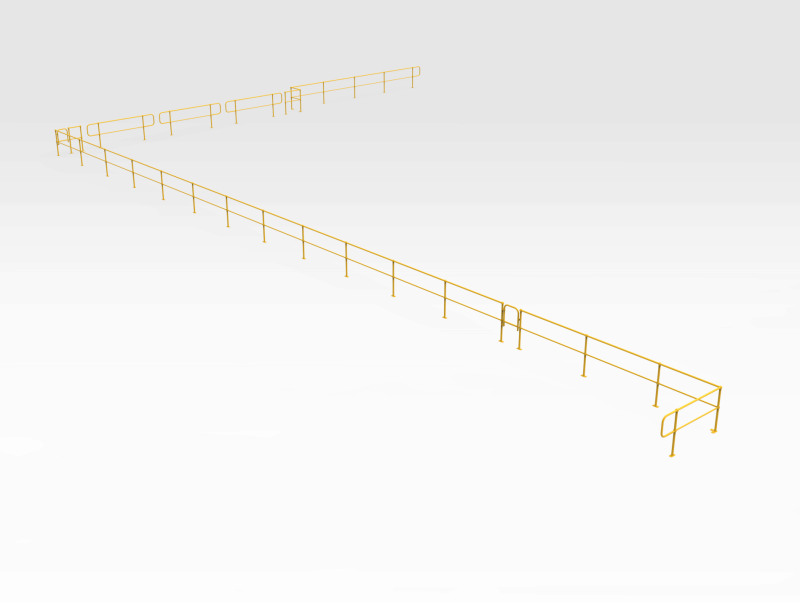The image depicts a yellow metal guardrail or railing, designed in a 3D art style and resembling the shape of an S or Z. The guardrail features a grid-like pattern and is seated on a plain white background that transitions into light gray hues as it moves upwards. This structure appears to function as part of an empty line queue, possibly for an amusement park, and is shown stretching from the bottom right corner of the image towards the top center. It consists of various segments connected by poles staked into the ground at regular intervals, likely every eight feet. The image creates a sense of depth, with the yellow guardrail extending into the distance, emphasizing its long length and continuous nature. The overall simplicity of the scene, combined with its computer-generated appearance, highlights the structure against the stark background.